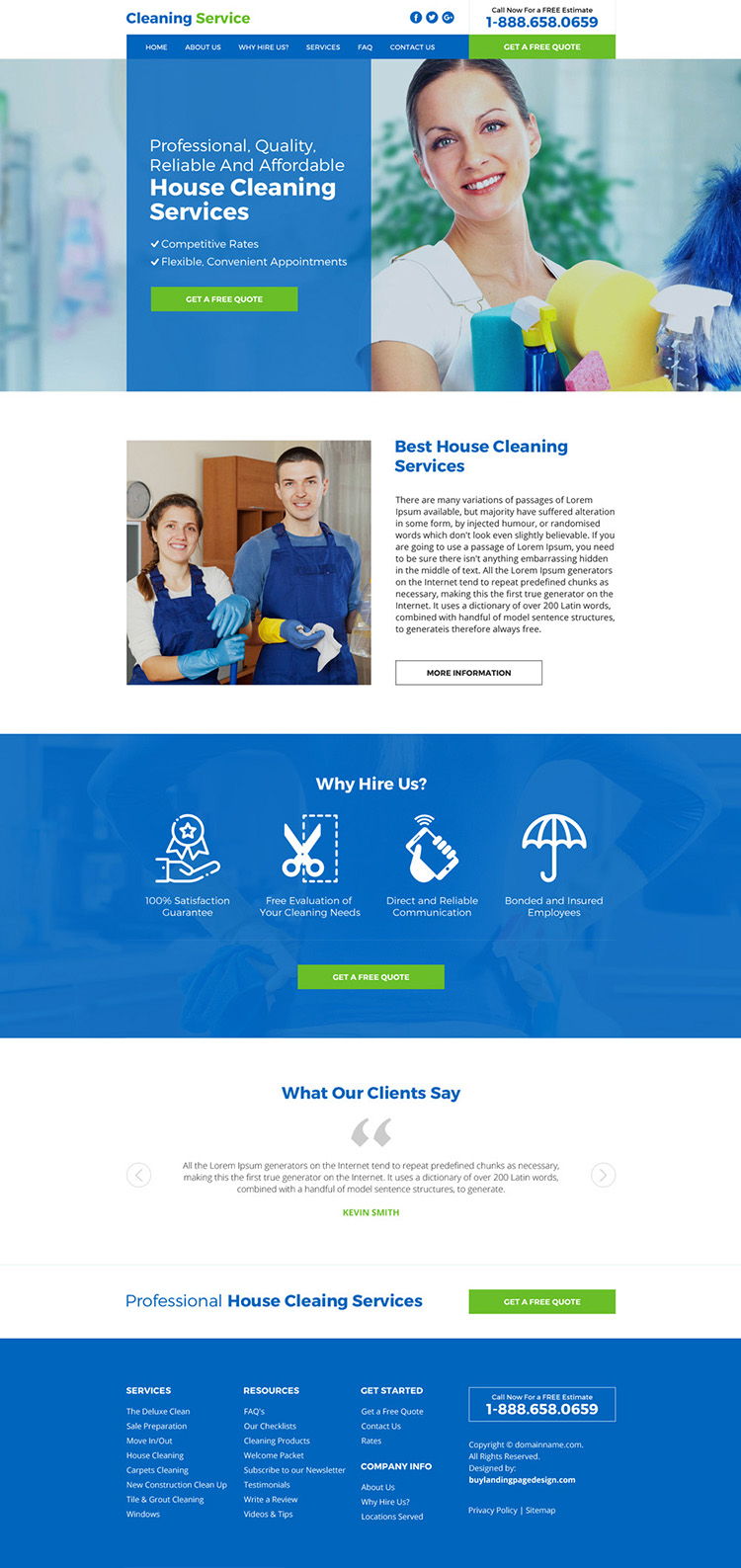This website appears to be for a professional cleaning service. The name of the service is not mentioned. In the top left corner, it says "Cleaning Services." To the right, there are social media icons for platforms such as Facebook, followed by a contact phone number, presumably 1-800-638-0659.

Below the header, there are navigational links for different sections of the website. The main banner reads, "Professional, Quality, Reliable, and Affordable House Cleaning Services." There are several features listed with check marks, though the text is too small to discern. Underneath, a prominent green button is displayed, though its purpose is unclear.

To the right of this section, there's an image of a house cleaning woman dressed in a white shirt, holding an array of cleaning supplies. She has dark brown hair. Beneath this image, the text claims, "Best House Cleaning Service."

To the left, there's another picture featuring a man and a woman, both equipped with rubber gloves and aprons, also holding cleaning supplies. Below these images, a section titled "Why Try Us" provides various links explaining the benefits of choosing this cleaning service.